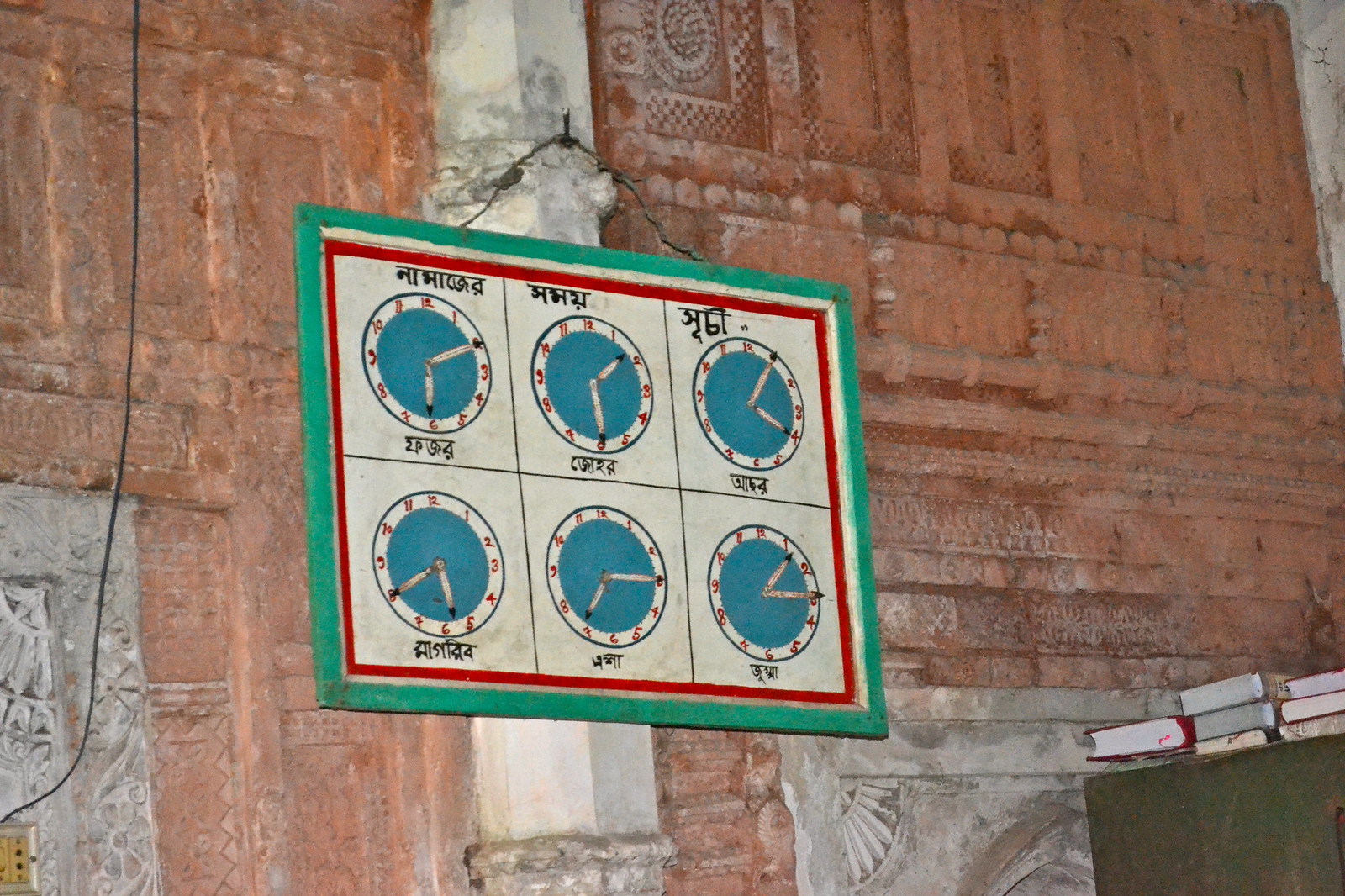This photograph captures a poster affixed to a pillar within a severely deteriorated and aged building interior. Both the poster and the structure are showing significant signs of wear and decay. The poster is segmented into six sections, each featuring a clock face set to a different time, and accompanied by labels written in what appears to be an Asian language, likely Hindi. Each clock face corresponds to a particular activity, suggesting a timetable for various tasks. Despite the industrial worksite implications of the schedule, the building itself exhibits elements more characteristic of a historical, possibly religious or cultural, edifice, evidenced by the intricate stone carvings adorning the walls. The juxtaposition of the modern, albeit worn, poster within such a venerable setting creates a striking contrast, blending elements of past and present.